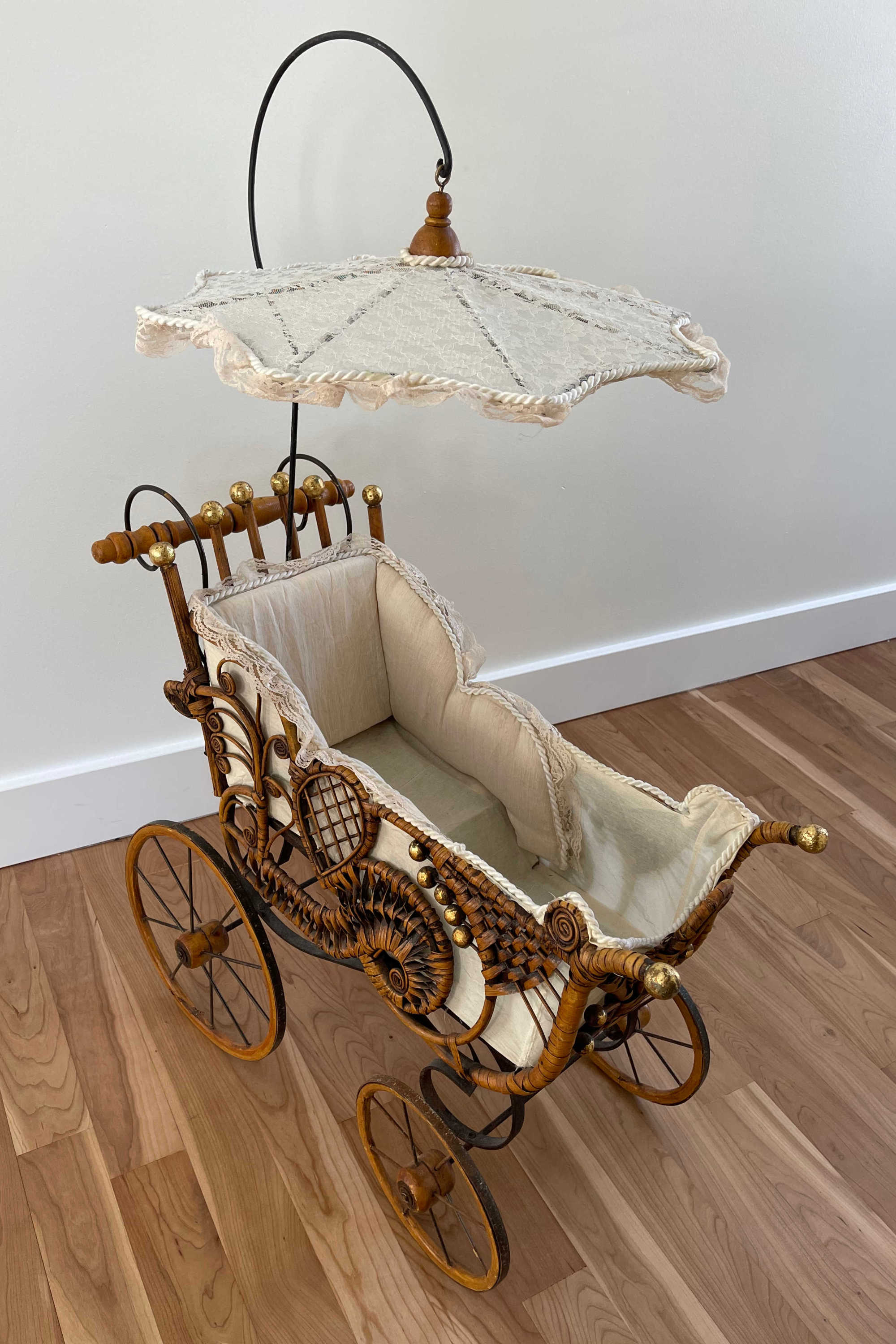This detailed photograph features an intricately designed, vintage-style baby carriage stroller situated indoors on a laminated wood floor. The stroller, resembling those from the Victorian era, showcases an old-world design crafted mainly out of wood, with a rich caramel brown hue, which contributes to its antique charm. 

The carriage boasts ornate side decorations with artistic carvings and patterns, including leaf-like and wicker basket elements, creating a sophisticated, old-fashioned aesthetic. The structure includes a pair of large rear wheels and smaller front wheels, both wooden with metal plating around the edges. These wheels lend an authentic, aged look to the piece.

A distinctive feature is the white, cloth umbrella on top, attached to a black wire frame with gold-tipped poles. This umbrella, adorned with braided and lace trim, provides shade and completes the carriage’s aesthetic. Inside, the stroller is lined with a plush, white pillowy surface, offering comfort and a luxurious feel. The interior also features intricate trimming, enhancing the stroller's delicate and refined appearance.

Overall, this baby carriage expertly combines an antique look with new-like condition, making it reminiscent of a cherished family heirloom or a premium collectible item.